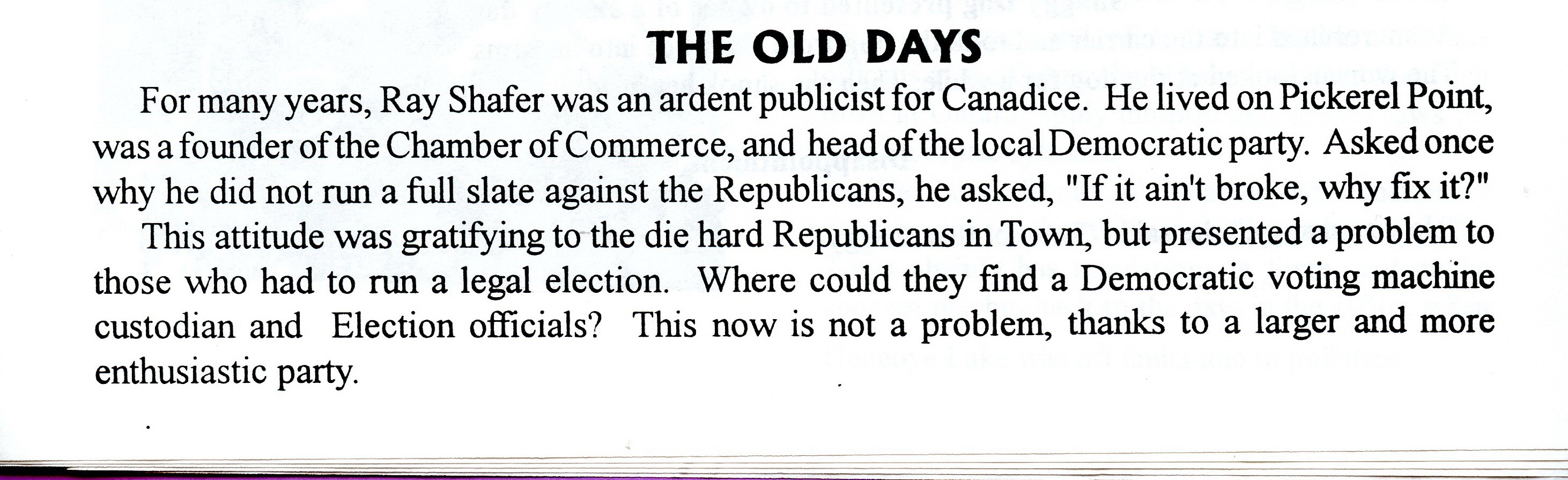The image shows a scanned piece of paper with a small passage printed in Times New Roman font on a white background. The title of the passage, "THE OLD DAYS," is prominently displayed in bold black letters. The text reads: "For many years, Ray Schaefer was an ardent publicist for candidates. He lived on Pickerel Point, was a founder of the Chamber of Commerce, and head of the local Democratic Party. When asked why he did not run a full slate against the Republicans, he replied, 'If it ain't broke, why fix it?' This attitude was gratifying to the diehard Republicans in town but posed a problem for those running a legal election. Where could they find a Democratic voting machine custodian and election officials? This is not a problem anymore thanks to a larger and more enthusiastic party." The paper appears to have other pages underneath it, suggesting it is part of a larger document.